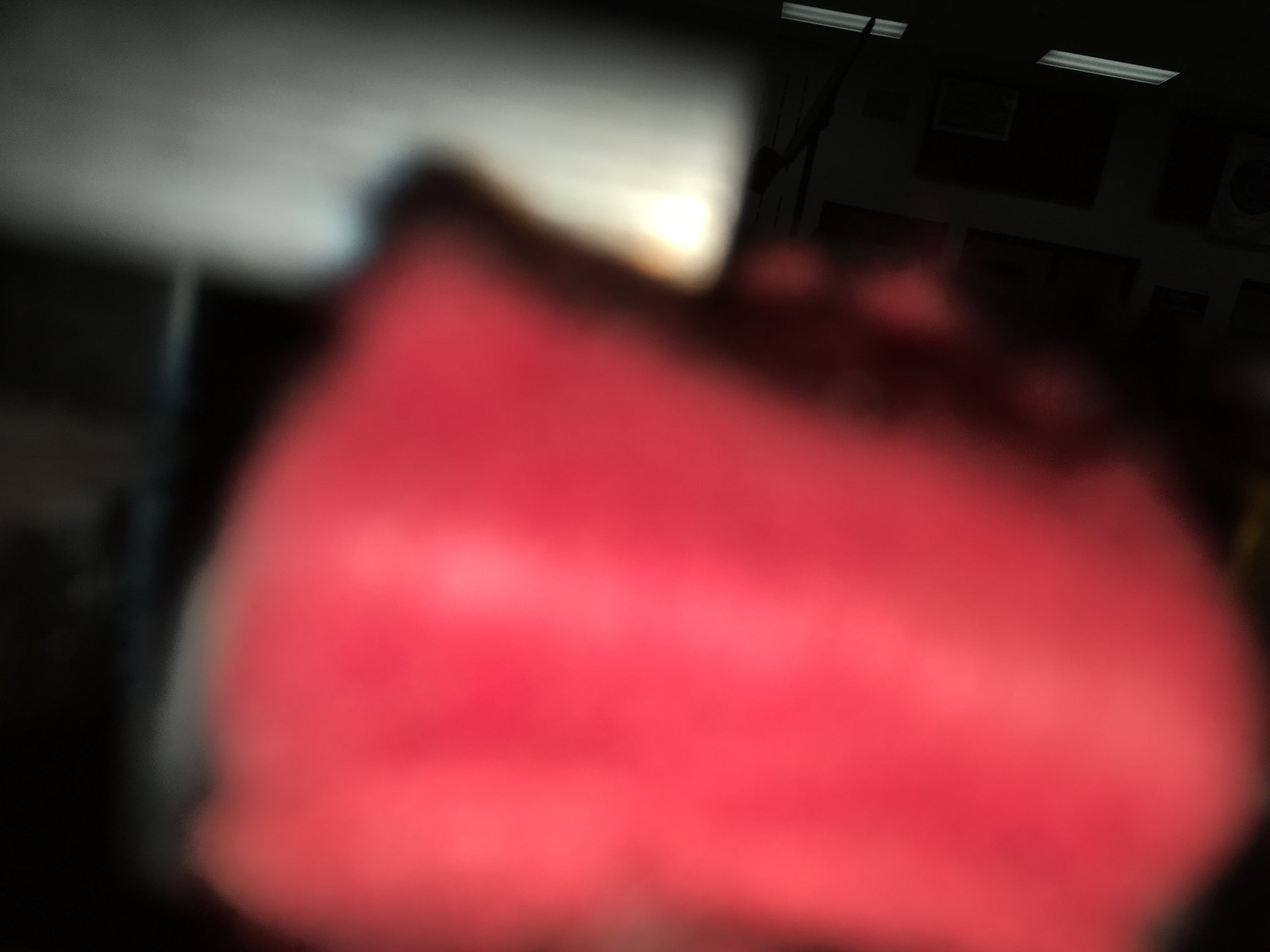This is a color photograph characterized by an indistinct and close-up perspective, shrouded in darkness and blurriness. Dominating approximately 50% of the central portion is a large, blurry red object with a rounded edge that stretches nearly across the entire image. The upper part of this red object, partially obscured in shadow, displays some small notches or points. Behind this red form, there is a blurry, rectangular white object, faintly illuminated along its right edge. A thin, greyish line extends from the bottom of this white shape, suggesting it could be a sign, although no writing is discernible. The backdrop of the image is predominantly black, with two small, broken, diagonal lines in the upper right corner, which might be fluorescent lights seen from a distance.